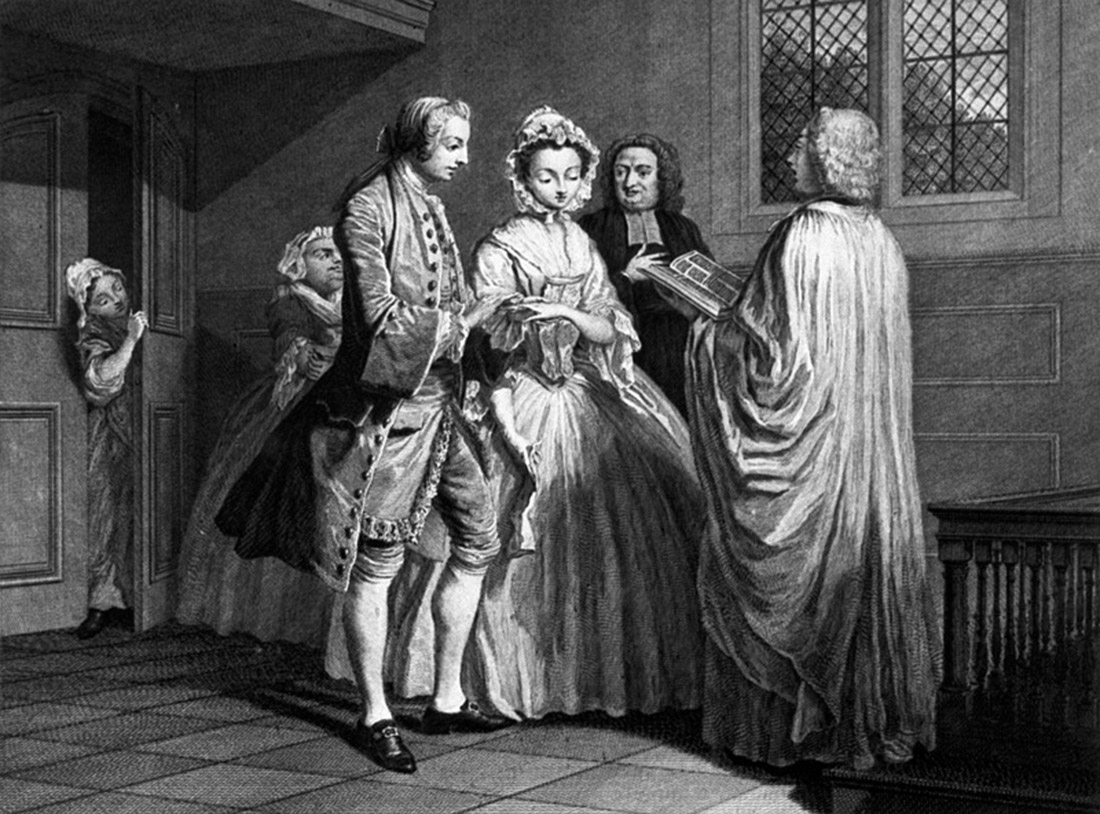This black and white sketch depicts what appears to be an old-fashioned wedding scene, likely from the era of the early American presidents. The men in the image exhibit hairstyles typical of that period, with their hair curled at the sides and pulled back, sometimes extending slightly longer. The central figure, presumably the groom, is dressed in knee-length breeches, tall socks, and a formal dress coat, adhering to the fashion of the time.

Next to him stands the bride, distinguishable by her voluminous dress, which is tightly fitted at the top and flares out widely at the bottom. She holds the groom's hand, symbolizing their union. To her right stands an individual clad in black, possibly a bridesmaid or another attendant, while a figure in front of the couple holds an open book, suggesting he is the officiant presiding over the ceremony.

In the background, a few more figures can be seen, likely guests or members of the wedding party, adding to the solemn ambiance of the setting. The ceremony appears to be taking place in a formal venue such as a church or city hall, indicated by the tiled floor, doors on the left, and a table and windows visible in the top right corner of the image.